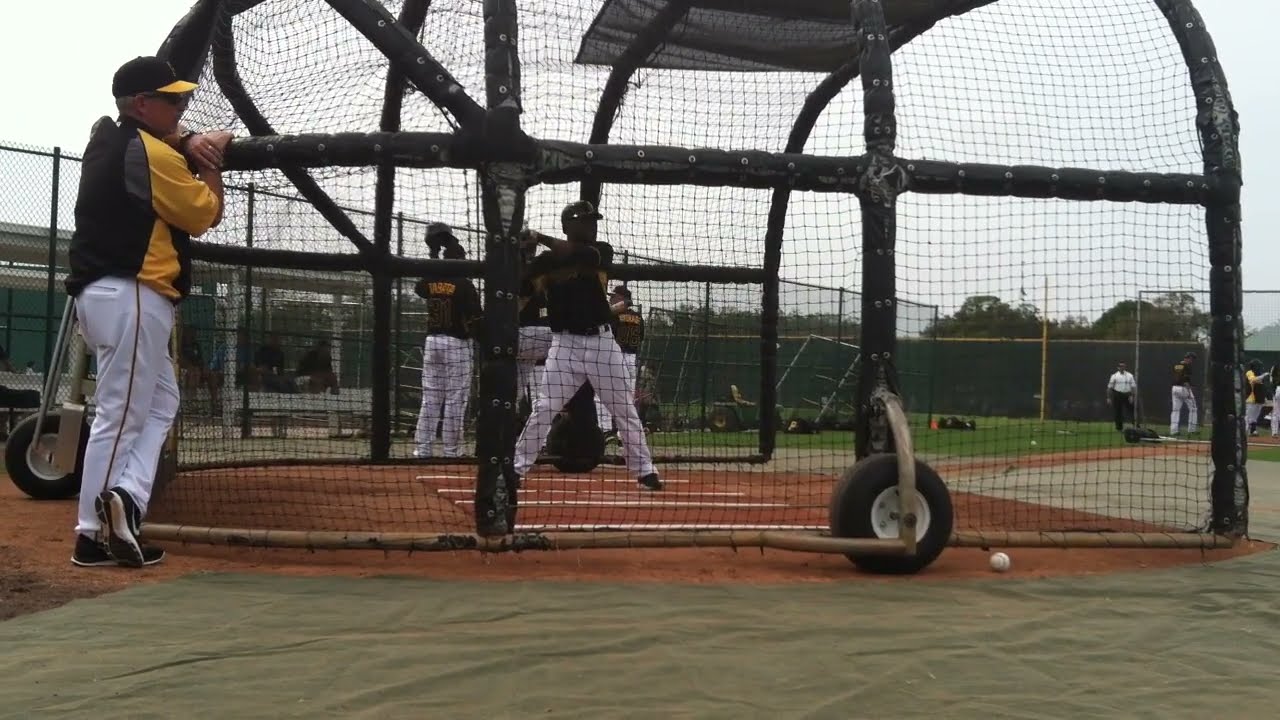Inside a baseball park during practice, a photographic image captures a detailed scene set against an overcast, gray sky. At the center of the frame, a player in a black jersey and white pants sits inside a movable batting cage, a sturdy metal structure with netting designed to contain errant balls and protect spectators. The batter appears to be holding a bat, poised to swing. Behind him, a group of team members dressed similarly in black jerseys and white pants is gathered, observing intently.

To the left of the cage, a figure in a distinct black and yellow jacket and matching baseball cap, along with white pants adorned with red striping, leans on the netting, closely watching the practice. In the top right section of the photo stands a man in a white shirt accompanied by more players congregating nearby.

The setting is rich with details: green grass underfoot transitioning to the brown dirt of the infield lined with white stripes. Beyond the outfield fence, a row of trees and hints of distant mountains frame the backdrop. Fencing and a green tarp add to the sense of being in a professional practice environment. The overall scene captures the focused atmosphere of a baseball team's practice session, highlighted by elements of their uniform and the readiness of their equipment.